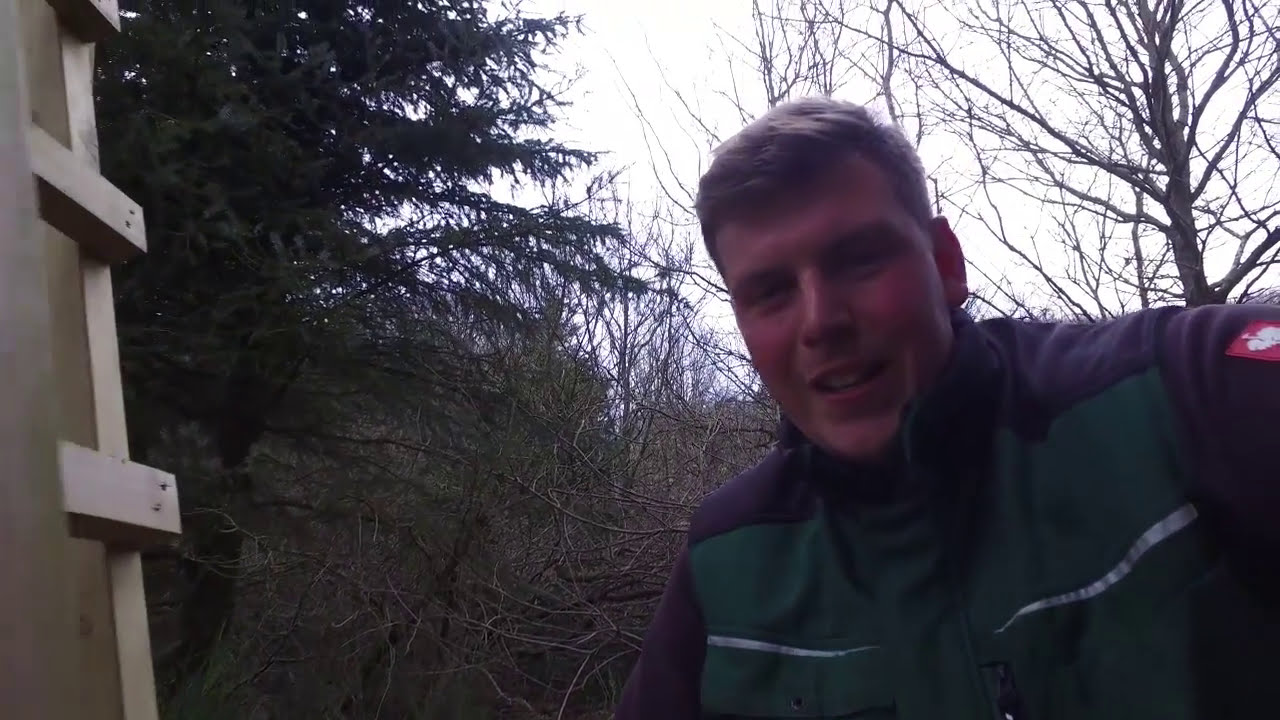In this outdoor selfie, a man with short dark hair is smiling at the camera. He is positioned in the lower right-hand corner of the image, wearing a green jacket with black shoulders and sleeves, adorned with a white spade insignia on the arm and silver stripes across the chest. The setting appears to be during the colder months, possibly fall or winter, as the trees behind him are barren, devoid of leaves. To the left, a wooden ladder leans against a structure, and an evergreen tree adds a splash of color against the otherwise stark backdrop. The lighting is backlit, casting shadows on his face and giving the image a dim, overcast atmosphere.